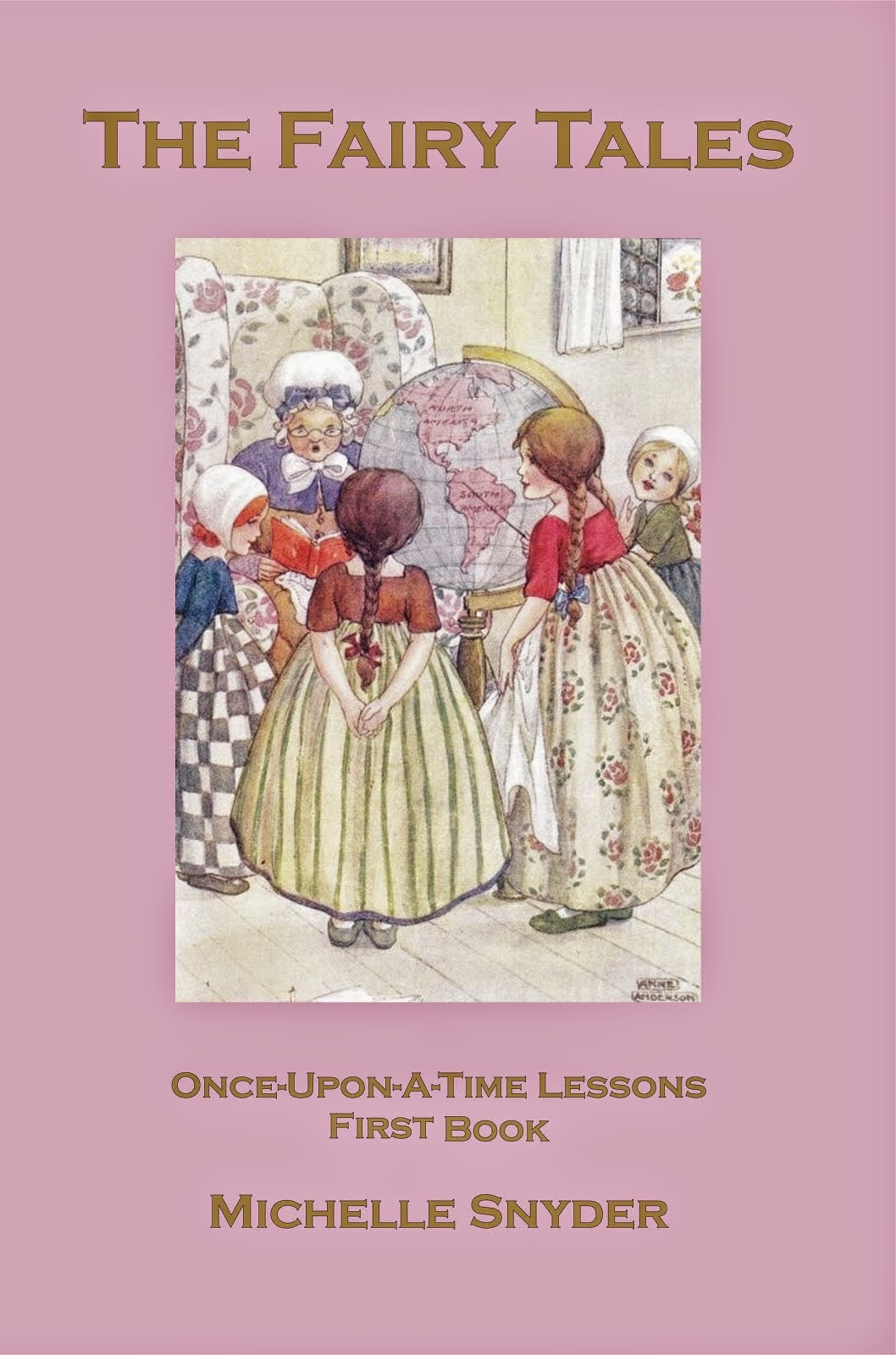This book cover features a light pink to mauve background with the title "The Fairy Tales" prominently displayed at the top in small caps and gold-colored text. Below the title, an illustration takes up most of the book cover, showing an elderly woman with glasses, wearing a white bonnet and a white bow, seated in a flowered wing-back chair. She holds an open red book and is reading to four little girls, all dressed in dresses, with two of them wearing bonnets. Next to the elderly woman is a large globe depicting North and South America. The setting appears to be a cozy room, as suggested by a window with curtains in the background. Below the illustration, more gold-colored text reads, "Once Upon a Time Lessons, First Book," followed by the author’s name, "Michelle Snyder."